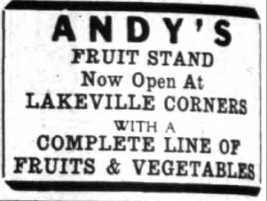The image presents a vintage advertisement likely clipped from a newspaper. It features a slightly rectangular, horizontally oriented layout with thick black lines running along the top and bottom edges. The central text, all in black, reads: "ANDY'S FRUIT STAND now open at Lakeville Corners with a complete line of fruits and vegetables." The word "ANDY'S" is rendered in bold, uppercase letters, while the rest of the text uses a thick, heavy font, possibly reminiscent of Times New Roman. The backdrop is a stark white, contributing to the vintage feel of the ad and suggesting it was typed, perhaps with a typewriter.